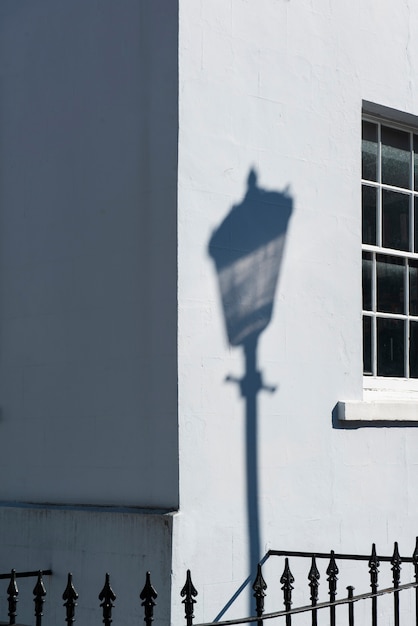The photograph, taken outdoors during the daytime, captures the corner of a stone or possibly stucco building. The left side of the building is a darker gray due to shadow, while the right side is a lighter gray or white and appears to be made of smooth stone. A window with small panes and a stone ledge is partially visible on the right side. At the bottom of the image, there's a black metal fence with spikes at the tips of its vertical bars. Dominating the scene is the shadow of an old-fashioned streetlamp cast against the building's wall. The streetlamp shadow features a pole with small protruding knobs and a conical lantern with a rounded top and a small point. The lantern section is semi-transparent, indicating where the light bulb would be. The overall composition highlights the interplay of light and shadow, adding a timeless, almost vintage atmosphere to the scene.